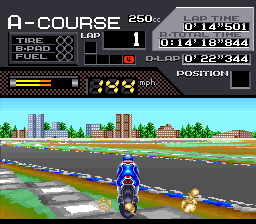The image depicts a screen from a computer game, showcasing a detailed scene of a motorcycle race. Dominating the foreground is a rider on a gray and black motorcycle, distinguished by a tail light and clad in a blue one-piece biking outfit paired with a blue and white helmet. The motorcycle and rider are positioned on a black racing roadway, bordered in bright blue, black, and white. A little walkway colored in white and gray highlights the surrounding green grass and dirt.

The backdrop features a skyline of buildings in varying shades of brown and gray, interspersed with lush green trees against a blue sky. Several of these buildings are detailed with white specks representing windows. Notably, there is a shorter brown building alongside a gray high-rise and a taller brown building flanked by more trees and brown structures.

At the top of the screen, a black box prominently displays game-related information in white text, such as "A-course, 250 CCs," along with "lap," "tire," "B-pad," and "fuel." Adjacent figures show lap times, total times, and position, while a black and brown checkered box below indicates the speed, set at 144 mph in yellow text. To the left, a black bar with neon yellow and orange accents appears illuminated, adding to the vibrant, game-like atmosphere. Additionally, the left side of the rider features a gold emblem, with another emblem on the right, enhancing the gaming interface aesthetic.